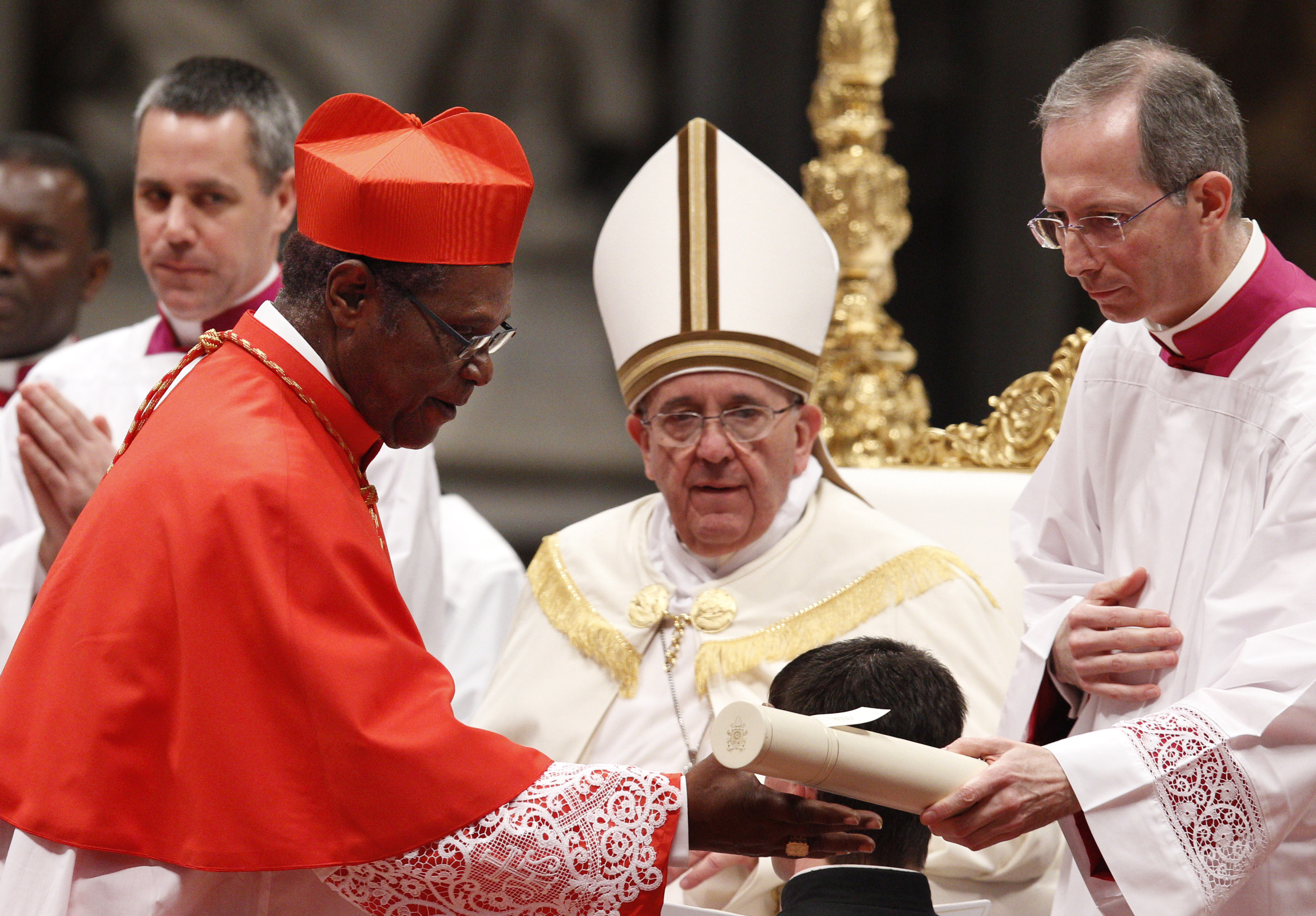The image depicts a religious ceremony, likely occurring inside a church, centered around what appears to be the Pope. The Pope is seated in an ornately decorated chair with white upholstery and golden ornamentation extending high above his head, featuring golden poles on the back legs. He is dressed in a white robe adorned with gold detailing and a tall white hat with tan and brown stripes down the edge and middle. Flanked on both sides by attendants in white robes with red collars and sleeve accents, the Pope is clearly the focal point of the scene. To the left of the Pope, there is a man in a bright orange robe with lace accents and an orange hat, who is receiving a cylindrical box with an open flap from one of the white-robed attendants. Additionally, three of the men on the right, who are also in white, are wearing glasses. On the far left side of the image, the partially visible head of an African American man can be seen. The background is a faded black, with a gold ornament noticeable near the Pope's head, adding to the solemn and regal atmosphere of this religious gathering.